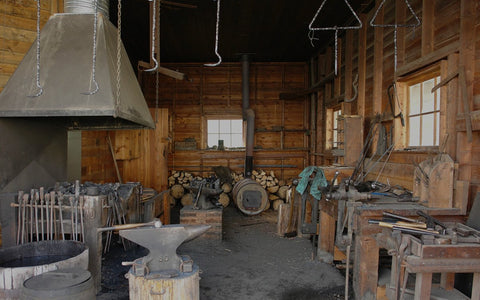The image depicts the interior of an old-time blacksmith's shop. Dominating the foreground, there's an anvil resting on a sturdy wooden stump, with a large hammer laid on top. The shop exudes a rustic charm with its natural wood surroundings, colored in various shades of tan and brown. On the bottom left side, an anvil is prominently placed, while the middle left features a forge filled with coal and a large metal hood above it, indicating a fire pit beneath. To the right, you'll find a well-organized workbench cluttered with various blacksmithing tools, and a vise is mounted on its edge. Hanging from the ceiling are chains and hooks, likely used by the blacksmith when working near the fire. A metal barrel, likely repurposed into a forge fireplace, stands out with its black stove pipe curving toward the roof. The back of the shop is lined with logs and wooden structures, reinforcing the shop’s earthy and utilitarian atmosphere. Hues of blackish gray, green-gray, green, walnut wood stain, and blue subtly enhance the overall aesthetic of this industrious setting.